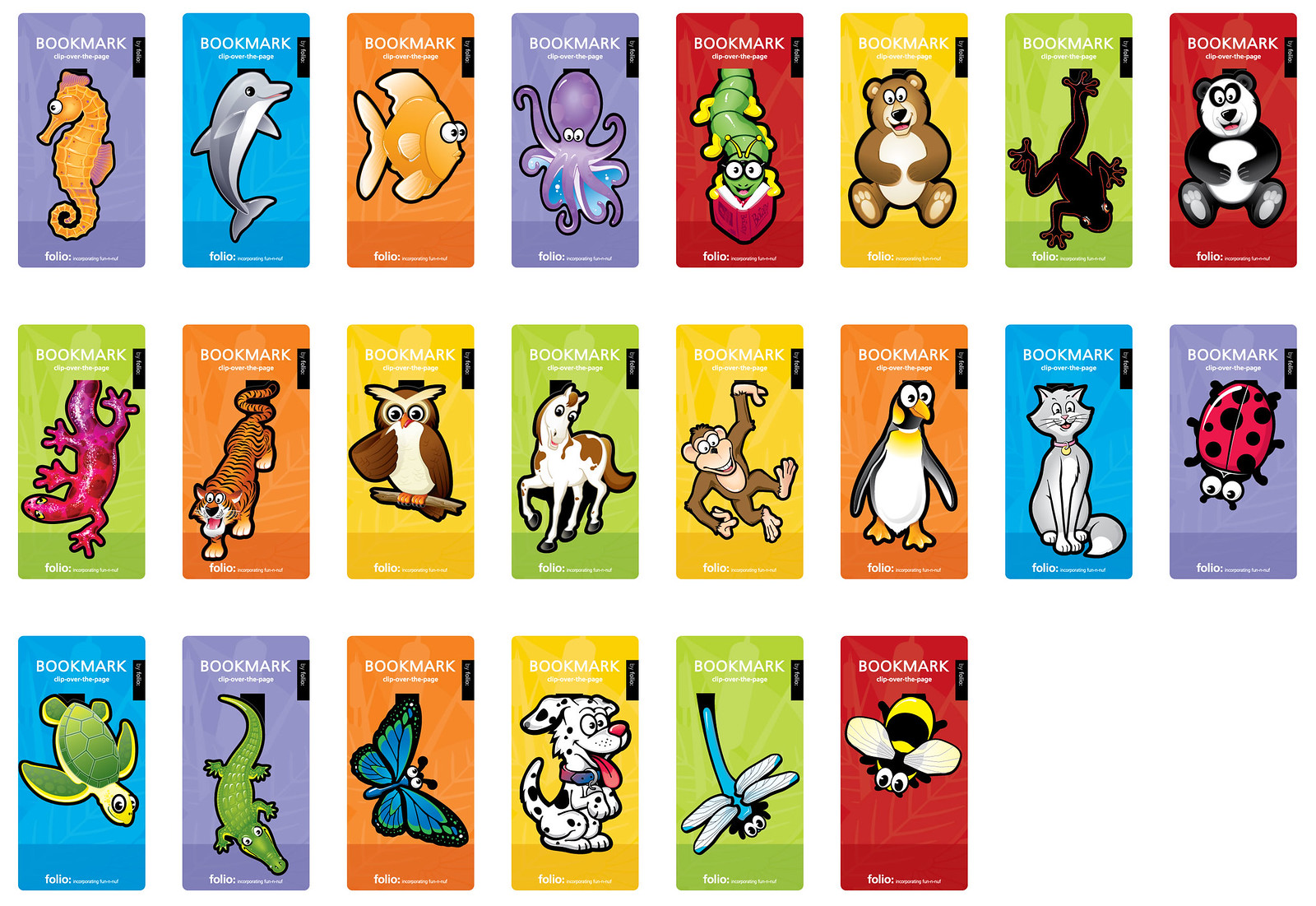This image showcases a vibrant series of 22 bookmarks arranged neatly in three rows against a solid-colored background, tailored for children. Each bookmark features a cute, cartoon-like animal with thick black outlines. The animals include a seahorse on a purple background, a dolphin on a blue background, a goldfish on an orange background, a purple octopus on a purple background, a caterpillar reading a book with glasses on a red background, a bear on a yellow background, a black frog on a green background, a panda on a red background, a pink gecko on a green background, a tiger on an orange background, an owl perched on a branch on a yellow background, a white and brown-spotted horse on a green background, a monkey on a yellow background, a penguin with large eyes on an orange background, a gray cat with a collar on a blue background, a ladybug on a purple background, a sea turtle on a blue background, an alligator on a purple background, a blue butterfly on an orange background, a Dalmatian dog with a collar on a yellow background, a blue dragonfly on a green background, and a bee on a red background. The top two rows contain eight bookmarks each, while the bottom row has six. Each bookmark prominently features the word "Bookmark" in bold white text at the top, with some smaller, unreadable white text below it and a tiny black bar containing another indiscernible white detail in the upper right corner.